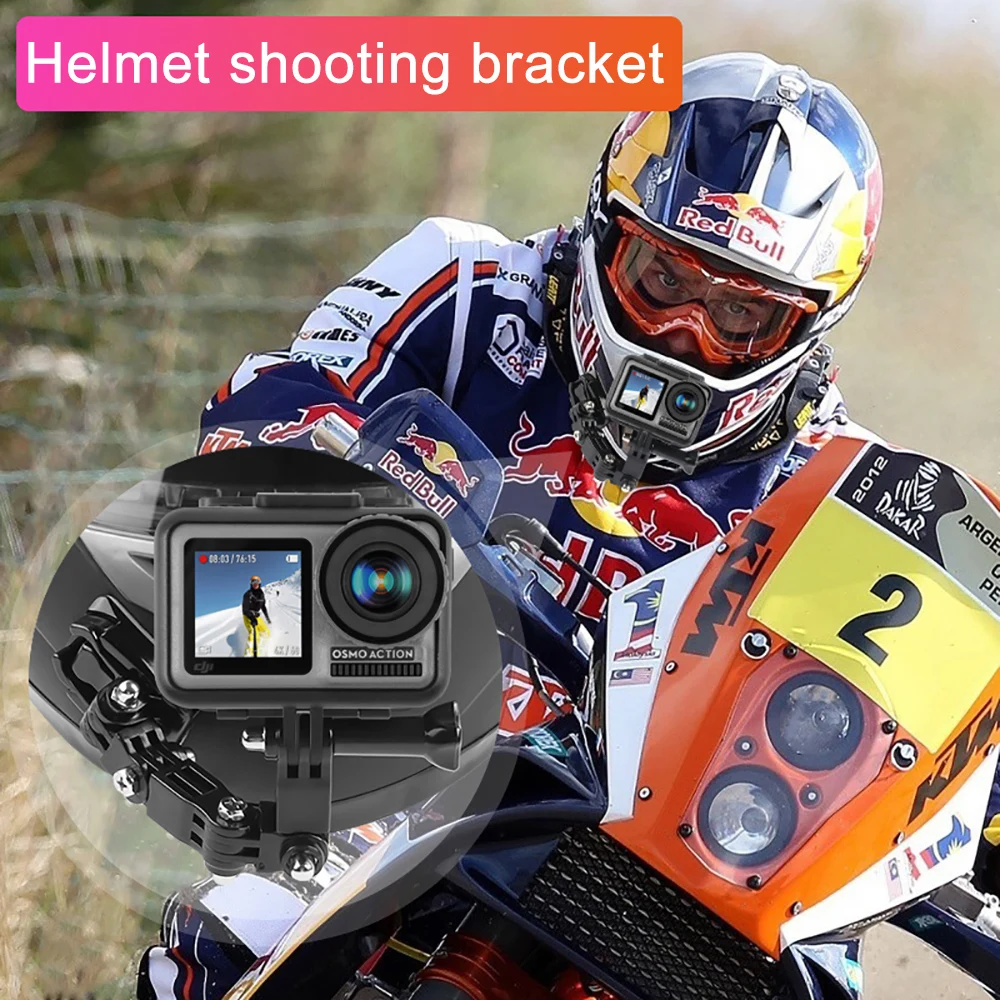This image showcases a dirt bike rider, likely sponsored by Red Bull, who is fully geared in a red, white, and blue racing uniform adorned with various advertisements. The rider is mounted on an orange motorbike, poised to ride straight ahead, with an intent expression visible beneath his helmet. His helmet prominently features the Red Bull logo along with two facing red bulls at the top front, highlighted by his mirrored goggles. A key focus of the picture is the ‘helmet shooting bracket,’ as emphasized by the bold white text on a pinky-orange background at the top left of the image. This bracket appears to secure a camera, specifically an Osmo Action camera, to the chin area of his helmet. This detail is further highlighted by an enlarged inset circle at the bottom left, providing a closer view of the camera attachment, underscoring the advertisement’s purpose of promoting this practical accessory for capturing dynamic riding footage.